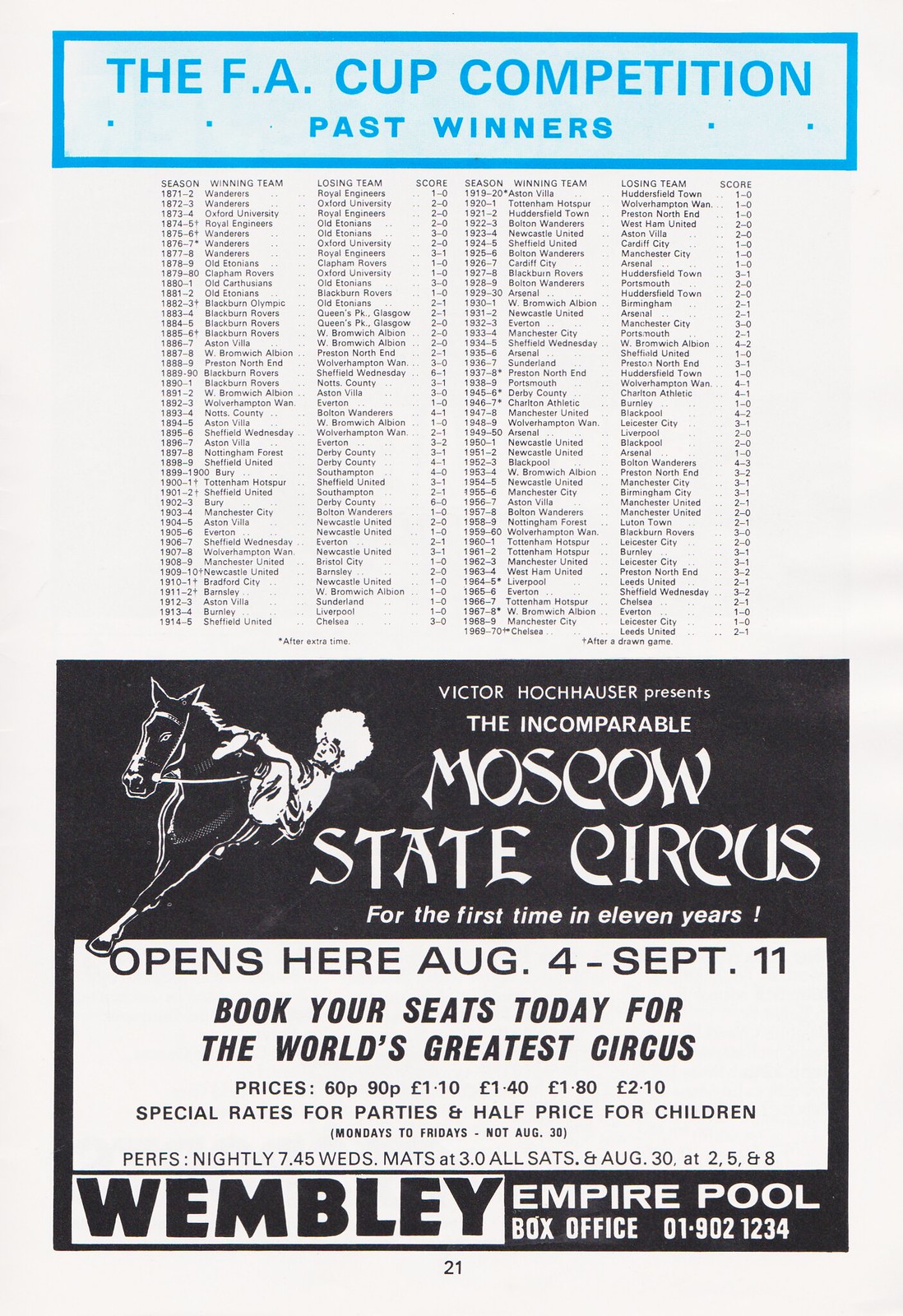The image depicts a page from a magazine, showcasing a detailed historical list of FA Cup competition past winners in a blue section at the top. The list spans from the 1871-72 season to the 1969-70 season, displayed in very tiny font, making it difficult to read. Below the list, there is an advertisement for the Moscow State Circus, presented by Victor Hochhauser. The advertisement features an image of a clown precariously riding a horse, drawn in a freehand style. It announces the circus's first appearance in 11 years, running from August 4 to September 11. The ad highlights ticket prices ranging from 60p to £2.10p, with special rates for parties and half-price tickets for children, valid Monday to Friday, except August 30. Tickets can be booked at the Wembley Empire Pool Box Office, with the provided phone number 0190-1234. The advertisement labels the circus as the world's greatest.